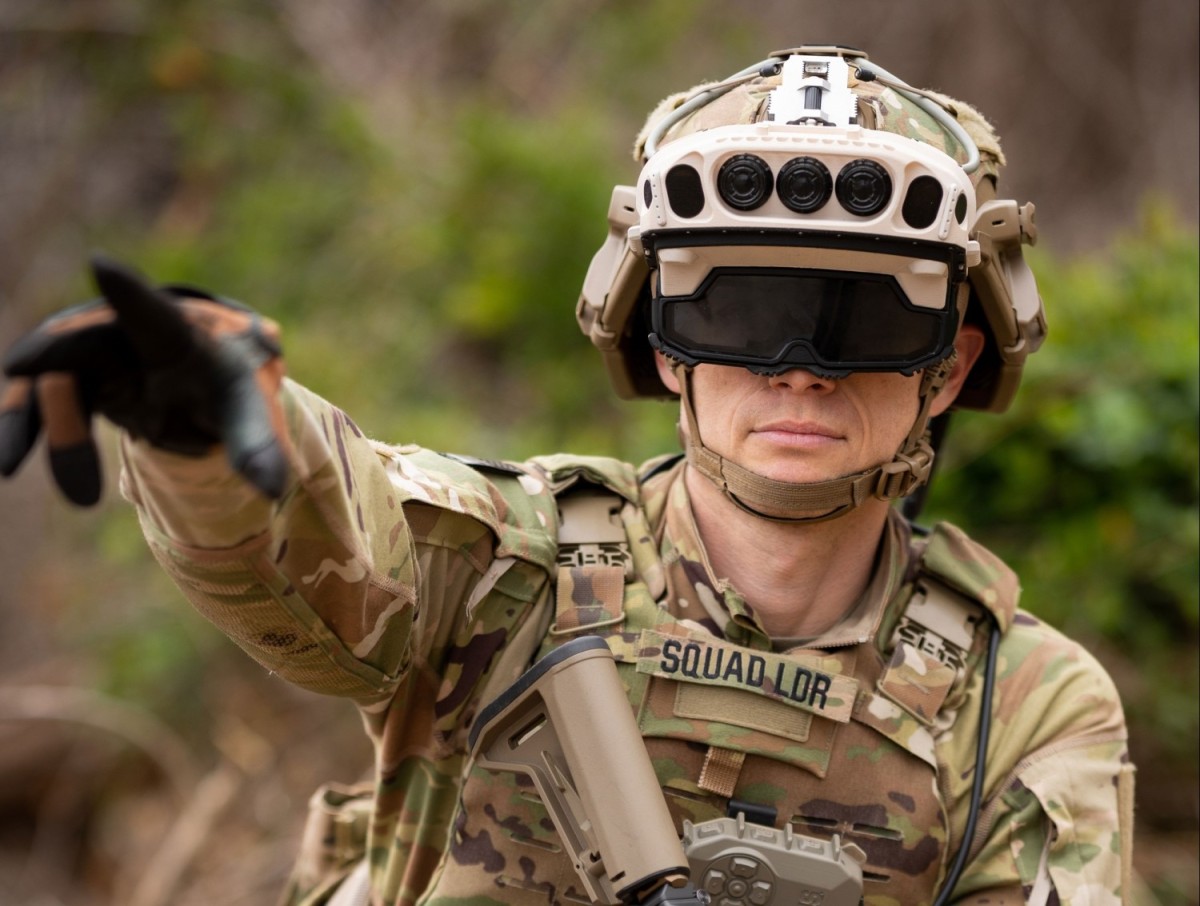This photograph captures a white soldier in a setting blurred with foliage, where trees and branches form an indistinct backdrop, ensuring the focus remains sharply on him. Dressed in brown, olive green, and tan camouflage fatigues, he carries the mark of authority with a chest patch labeling him as "SQUAD LDR." On his head, he wears a camouflaged helmet affixed with a white visor device, resembling multiple lenses akin to spider eyes, presumably for advanced visual capabilities or heads-up display. Beneath this complex apparatus, he shields his eyes with dark, sunglass-like protection. His chin strap secures the helmet firmly. He stands with his right arm extended and a gloved finger pointing forward, suggesting direction or command. The stock of his tan-colored rifle emerges from the bottom of the frame, hinting at his readiness and vigilance.